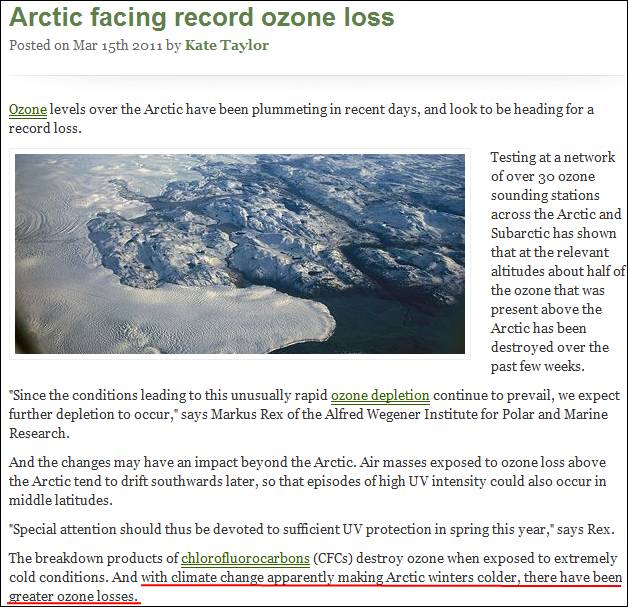A screen capture from a web article detailing significant ozone depletion in the Arctic is showcased. The headline at the top of the page reads, "Arctic Facing Record Ozone Loss," with the article being posted on March 15, 2011, by Kate Taylor.

The article begins by reporting that ozone levels in the Arctic have dramatically declined in recent days, with indications that they are heading towards record losses. Testing conducted at a network of over 30 ozone-sounding stations in the Arctic and subarctic regions reveals that approximately half of the ozone present at certain altitudes above the Arctic has been depleted over the past few weeks.

Further down, the article features expert commentary from Marcus Rex of the Alfred Wegener Institute of Polar and Marine Research, stating, "Since the conditions leading to this unusual rapid ozone depletion continue to prevail, we expect further depletion to occur." Rex also warns that the impact of these changes may extend beyond the Arctic, noting that air masses affected by ozone loss tend to drift southward. This can result in episodes of unusually high UV intensity in more temperate regions, necessitating heightened attention to UV protection during the spring.

The piece concludes by explaining that the breakdown products of chlorofluorocarbons (CFCs) are responsible for ozone destruction when exposed to extremely cold conditions. Climate change, which appears to be making Arctic winters colder, is contributing to even greater ozone losses.